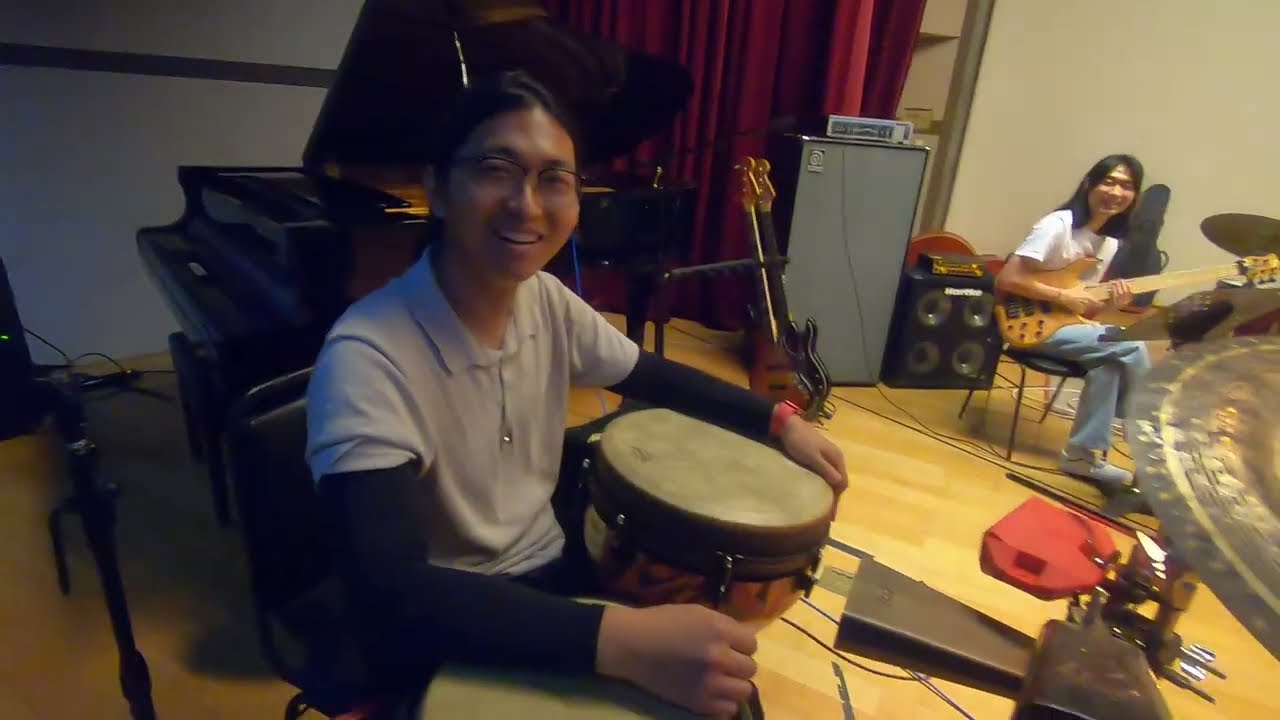In the image, a small group of Asian-origin musicians is staged for a performance. Centrally positioned, a man wearing a white polo shirt with a black long-sleeve shirt underneath and glasses holds a bongo drum, smiling warmly at the camera. In front of him, horizontally oriented cowbells and cymbals suggest he is a percussionist. To his right, a woman with long black hair, in a white shirt and blue jeans, cradles a brownish-tan guitar, her smile equally vibrant. Both are seated in black chairs.

A black grand piano with its top open rests behind them, unmanned. The stage is cluttered with numerous wires and various speakers, including a tall gray one with wires spreading out and a square-shaped black one. Directly behind the guitarist, an amplifier sits atop what appears to be a shipping box or suitcase. Additionally, the backdrop includes a red curtain and a segment of white wool further to the right. Scattered behind the musicians are a couple of other guitars leaning against a light gray speaker and what seems to be a guitar stand on the left-hand side. The scene suggests an intimate, possibly in-studio setting.